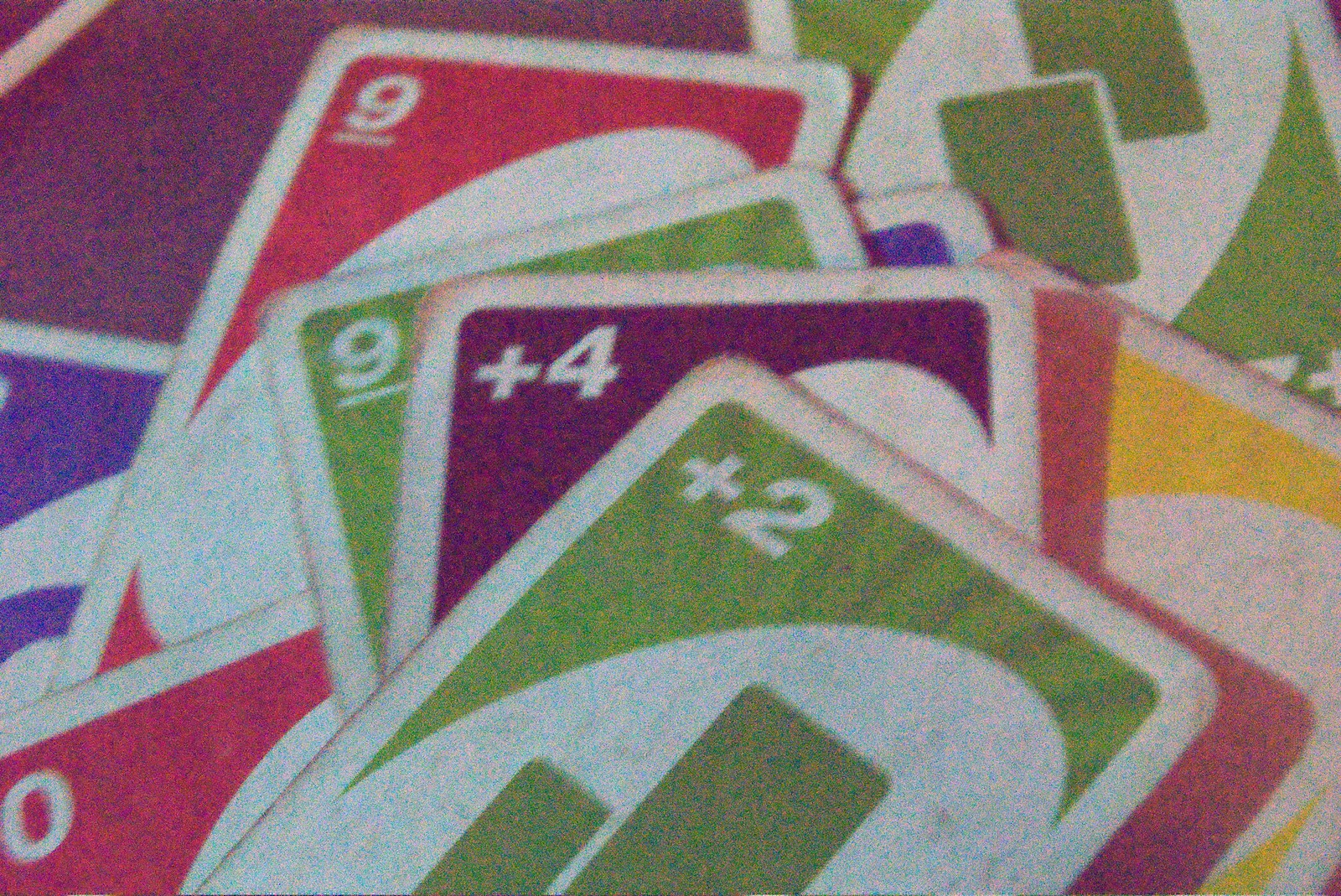The image depicts a slightly out-of-focus photograph in landscape orientation featuring an assortment of colorful cards, which appear to be part of a math game rather than standard playing cards. The cards are stacked haphazardly, showcasing a variety of hues and numerical values. The topmost card is green with two green rectangular bars and a white oval. It prominently displays a "plus 2" in white text. Immediately beneath it, a purple card shows a "plus 4." The third card down is another green card featuring an underlined number "9." The fourth visible card, which is pink, also bears an underlined number "9." To the left side of the stack, a separate card with a prominent "0" is visible, which could potentially be part of a "10." The cards are decorated with different patterns of rectangular bars, adding to their unique appearance. The overall composition suggests a game that involves numerical strategy or arithmetic.